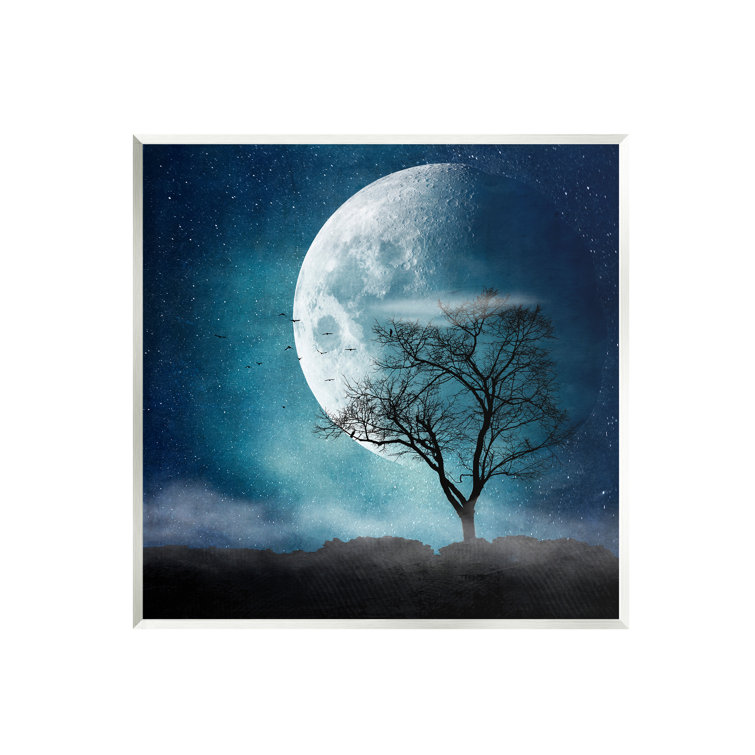The image is an artistic painting showcasing a captivating night scene. At its center is an enormous, beautifully detailed moon, prominently displayed slightly off-center to the right. This full half-moon features a brightly lit side with a subtle blue aura and a darker side that's still visible. Surrounding the moon is a starry night sky with numerous stars scattered throughout.

In the foreground, there's a striking silhouette of a barren tree, resembling a dogwood tree, with gnarled branches extending upwards. Below this tree, low-lying fog covers part of the jagged, rocky land, adding a mystical ambiance to the scene. Silhouetted against the moon are several small birds, appearing to fly away from the tree, their forms sharp against the moon's radiant glow.

The painting, possibly done on canvas, has a slight three-dimensional texture, enhancing its lifelike quality. The combination of the moon's luminescence, the serene yet eerie landscape, and the fine details such as the fog and the birds, make this artwork a mesmerizing representation of a star-studded nocturnal view.